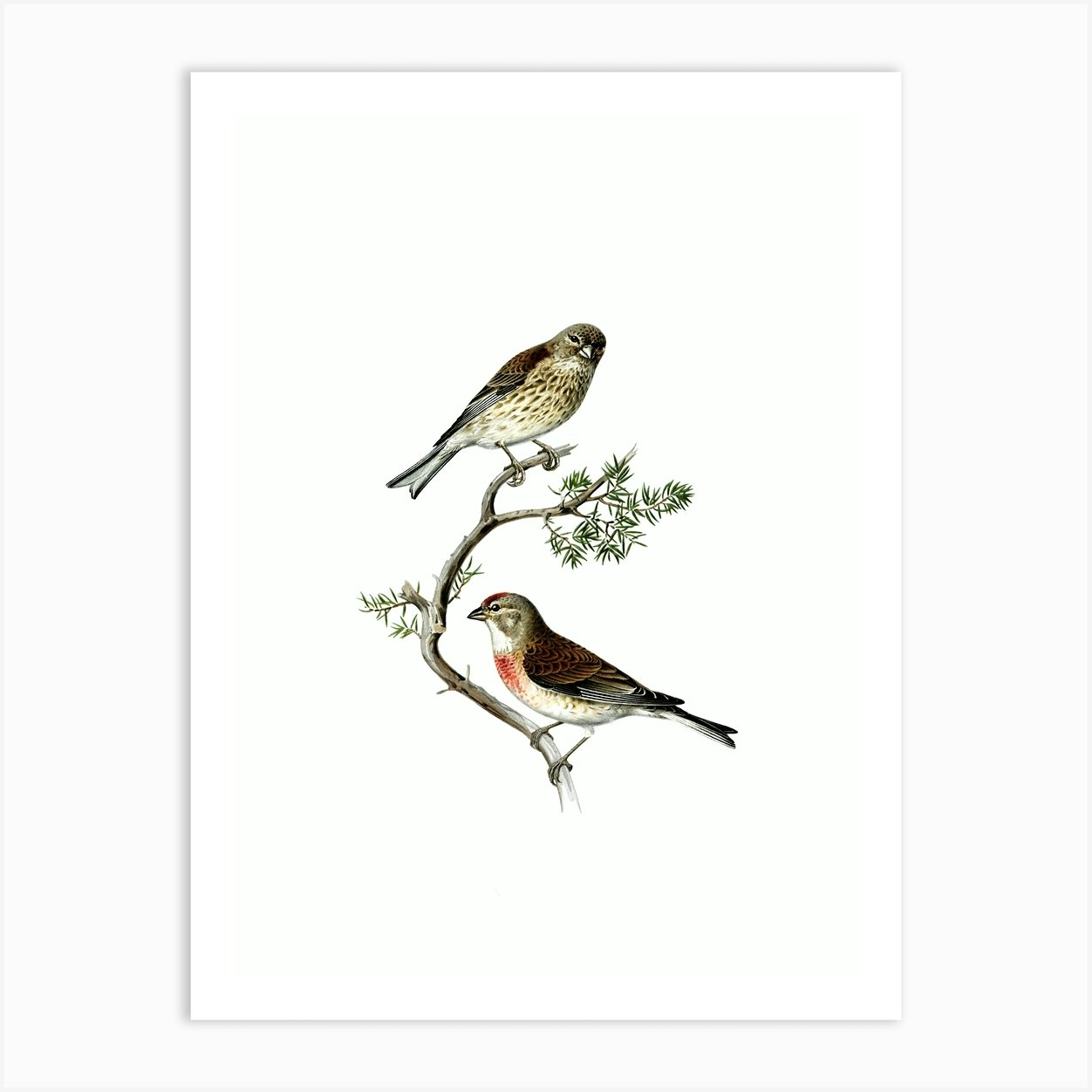This is a detailed and colorful illustration of two small birds resting on a rather bare pine branch, which is curved in a C-shape and adorned with sparse pine needles. The background is pure white, framed by a slightly brighter white border. The top bird is perched on the left side of a forked end of the branch, tilting its head to gaze directly at the viewer. This bird features a brown back and a light brown belly, with darker brown feathers giving it a textured appearance. The second bird, located at the bottom of the branch, is in profile and facing left. This bird is characterized by its brown wings and pointed tail, white belly with distinctive red marks, and closed beak. The intricate illustration showcases the meticulous rendering of the feathers, indicating a high level of detail and craftsmanship, although the artist remains unidentified.